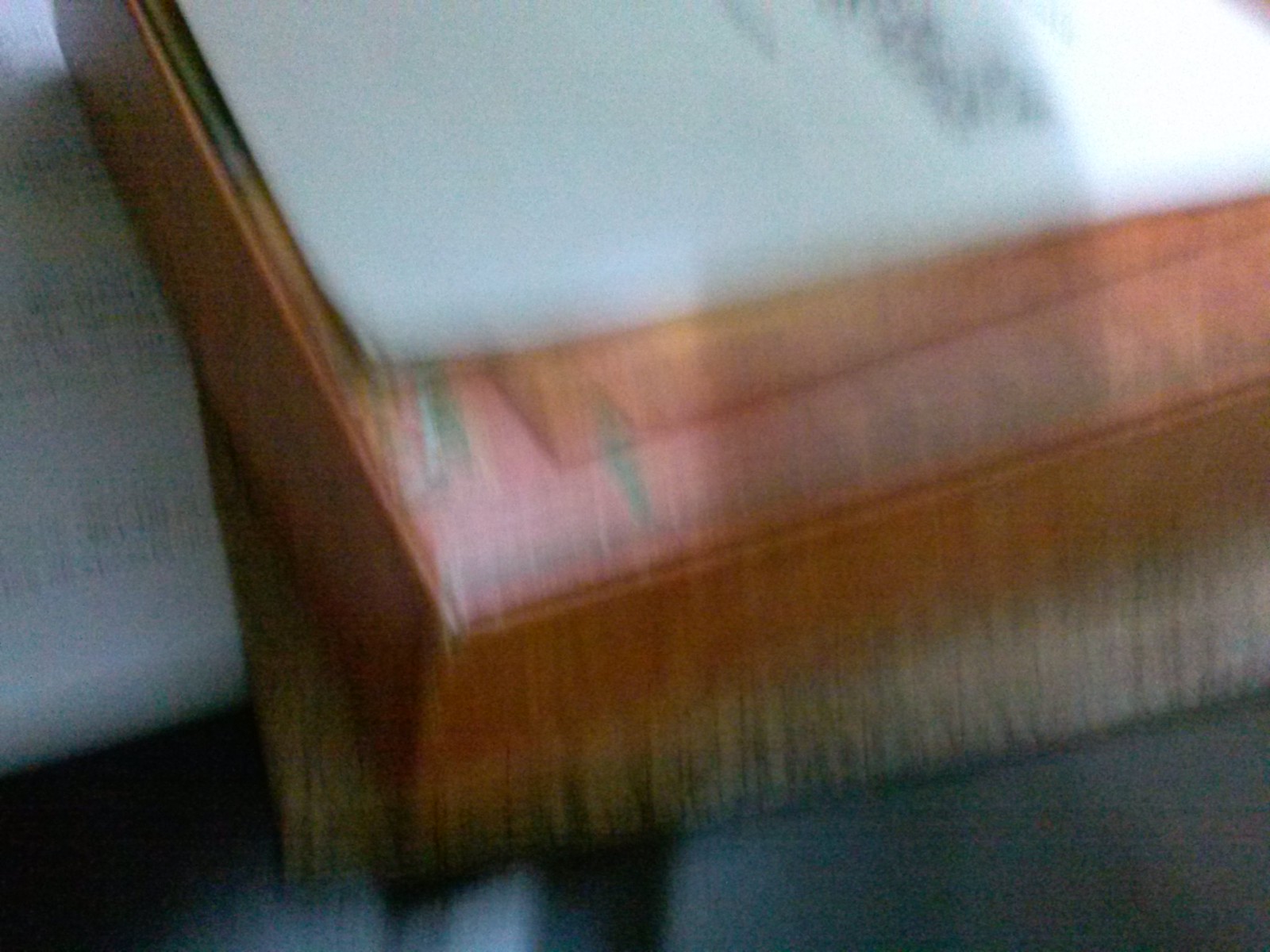The photograph appears to be an accidental capture, likely taken as someone removed their phone from their pocket. The image is noticeably blurry, with no clear subject in focus. Predominantly visible is the corner of a wooden table, suggesting the shot was taken from a low angle. On the surface of the table, there is a vague outline of a white piece of paper, though the blurriness obscures any specific details. The overall impression is of an unintentional and unfocused snapshot.